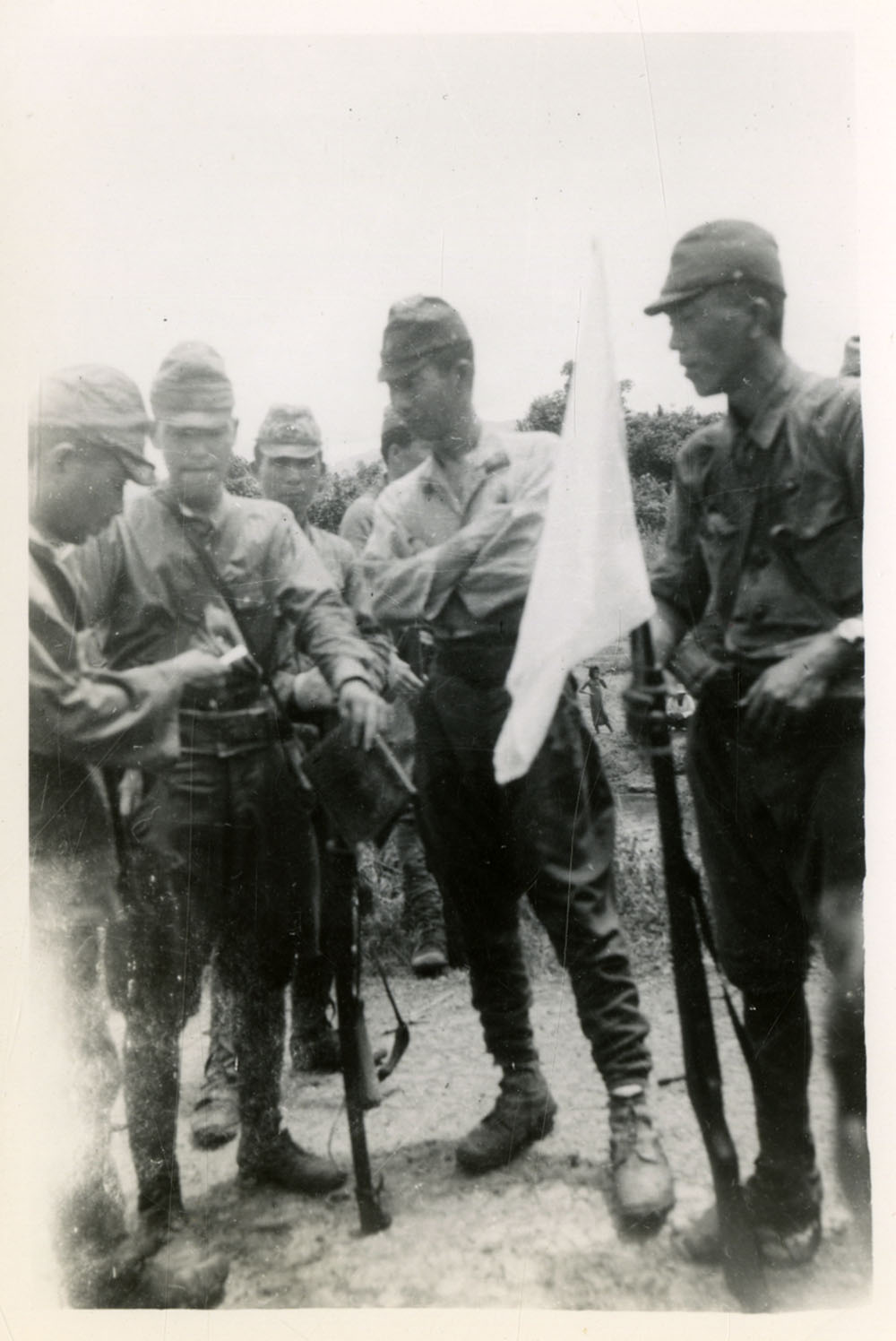This detailed black-and-white photograph from World War II shows five Japanese soldiers, four of whom are standing in a circle holding their rifles. The focal point of the image is the soldier holding a rifle with a white flag attached, indicating their surrender. All soldiers are dressed in World War II-era uniforms with buttoned shirts and caps. The soldier on the left appears to be examining a notebook, observed intently by two other soldiers standing close by. In the background, more Japanese soldiers can be seen milling around, contributing to the sense of a larger scene. The photograph, slightly faded especially in the corners, appears to be set on an island, evidenced by the trees visible in the background. This poignant image likely captures a moment towards the end of World War II when Japanese forces began surrendering to the Allies.